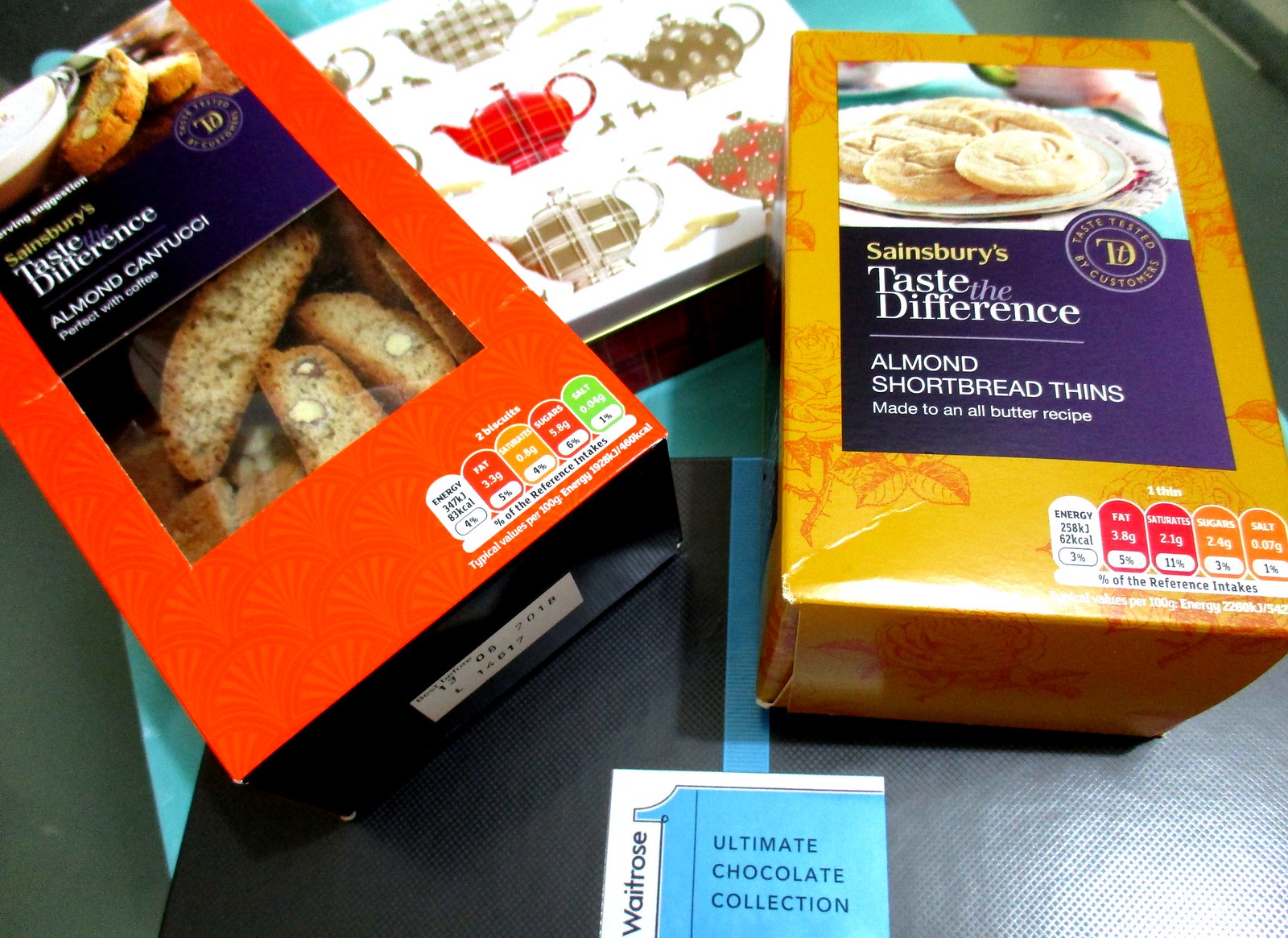The photograph depicts an assortment of gourmet food items arranged on a dark table. On the left is a red box of Sainsbury's Taste the Difference Almond Cantucci, featuring a transparent window that reveals the bread-shaped treats inside, ideal for pairing with coffee. To its right, there's a brown box of Sainsbury's Taste the Difference Almond Shortbread Thins, made to an all-butter recipe, with detailed nutritional information displayed on the bottom. Both of these boxes rest on a larger black box labeled "Ultimate Chocolate Collection" from Waitrose, adorned with a blue ribbon. Slightly to the left and behind them is a tin container embellished with various patterns of coffee or teapots, possibly containing more cookies or tea bags.